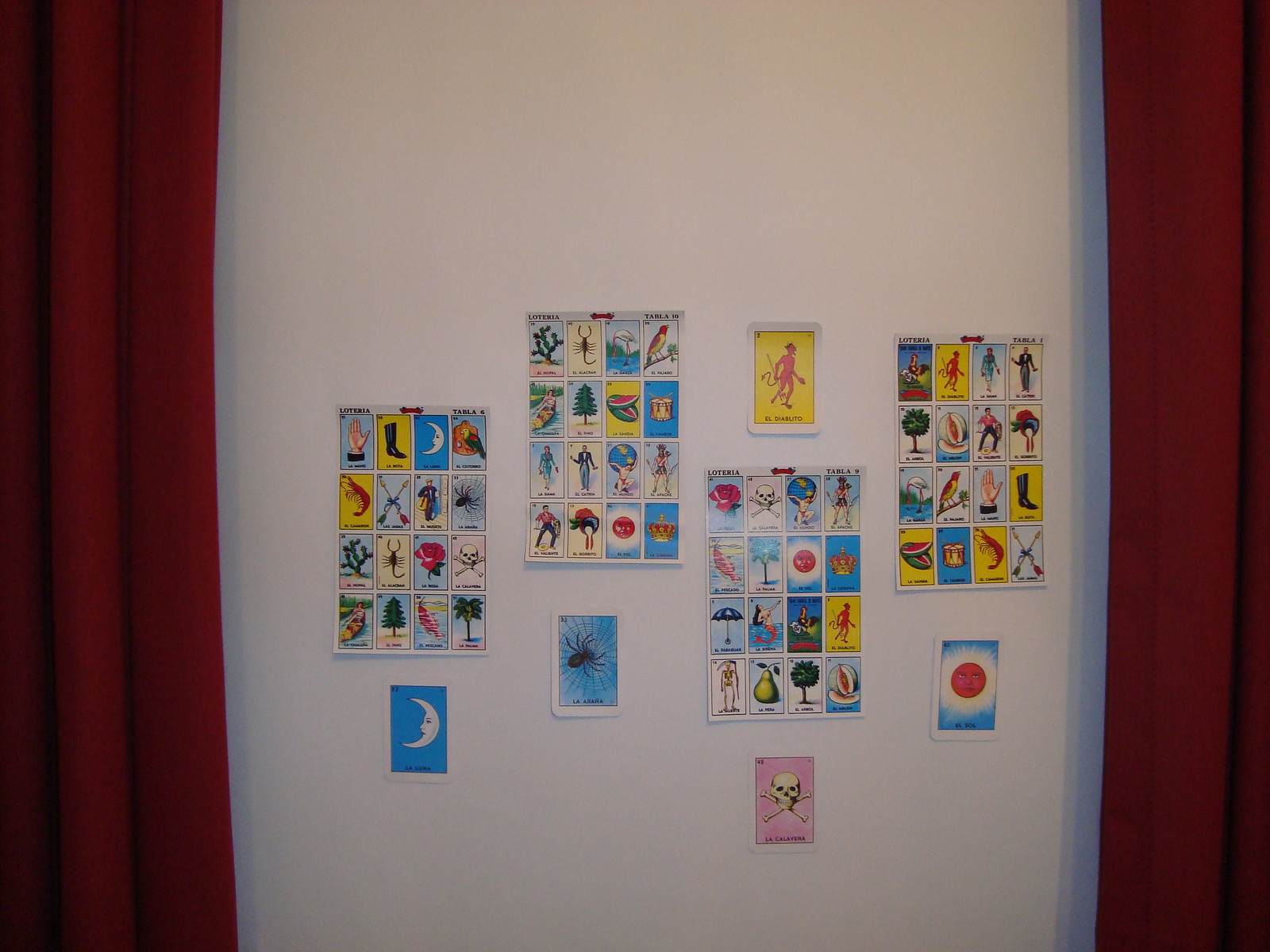A brightly lit room features a striking white wall adorned with vibrant decorations. Framing the wall are red curtains on either side, casting delicate shadows upon the pristine surface. Taped to this wall are numerous colorful images resembling tarot cards, exhibiting an array of vivid hues including reds and blues. These images depict various symbols and scenes: a hand, a moon, a scorpion, a tree, a rose, a skull and crossbones, a palm tree, a cactus, a prawn or lobster, and a group of people. In addition to the scattered individual cards, there are four large posters showcasing groups of these images. Among the separate cards, notable ones include a blue-backed card with a red sun emitting white beams, a pink card with a yellow background and a skull and crossbones, a blue-backed card with a black spider on a web, and a card featuring a white moon against a blue background.